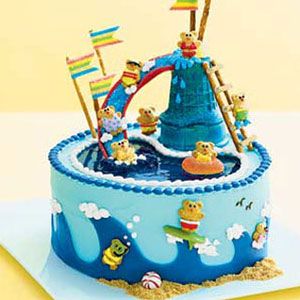This is a detailed image of a children's birthday cake, possibly intended for a child with a love for the beach or ocean themes. The cake, which seems perfect for both boys and girls, is primarily a light blue, aqua blue color, representing an ocean. Dark blue fondant waves, accented with air bubbles, rise from the base to the top, creating an underwater illusion.

At the base of the cake, there's a sandy texture, likely made from brown sugar, mimicking a beach. Decorative elements include little characters like teddy bears, some of which are depicted surfing and snorkeling along the edges of the cake. These teddy bears are intricately adorned, with one even wearing a red bikini.

On the top, the cake features a detailed pool scene, complete with a ladder leading up to a tower. From this tower, a water slide spirals down into the pool. There are several teddy bears involved in various activities: three sliding down the water slide, one standing at the top, one in the pool with an inner tube, one on the ladder, and one beside the tower. Additionally, blue, green, and red flags protrude from the top of the cake, adding to the festive and whimsical atmosphere. 

All these details sit against a backdrop of a white counter and a yellow wall, highlighting the vibrant colors and playful design of the cake.